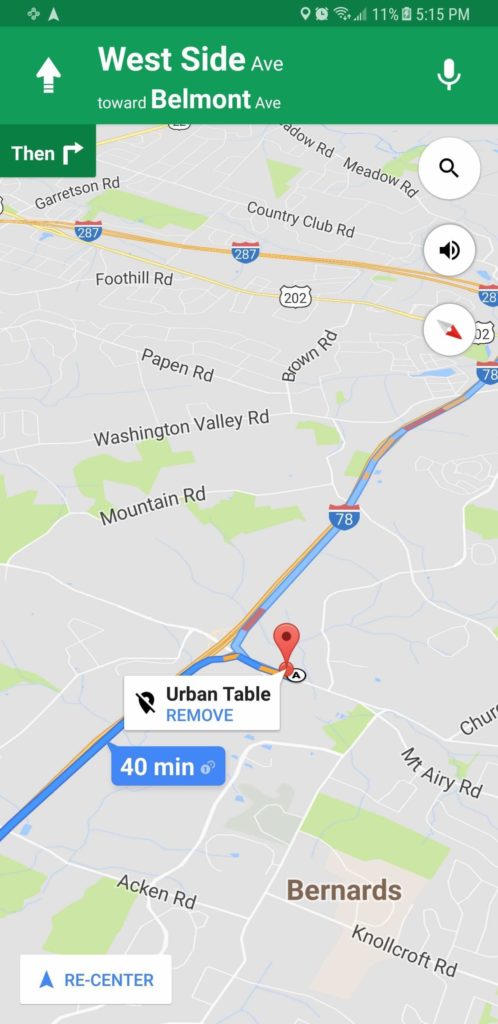The image depicts a navigation application interface on a smartphone. The upper part of the screen features a green header accompanied by a thin dark bar showcasing various icons in sequence: a directional arrow on the left, a location marker, an alarm clock, a Wi-Fi signal, mobile signal strength, an 11% battery indicator, and the time displayed as 5:15 PM. Below this, a wider, lighter green bar spans the width of the screen, displaying an up arrow with two dashes at its base and the text "West Side Avenue" in white, followed by "towards Belmont Avenue." A microphone icon is positioned to the right of this bar.

Beneath this section, there's a tab indicating the next navigation step: "then turn right," suggesting the image showcases a GPS-based driving application. The map displayed is in 3D, illustrating various roads and streets, prominently featuring Highway 78. A speech bubble connected to the highway mentions a travel time of "40 minutes." A marker labeled "A" identifies a location named "Urban Table." While the specific destination isn't explicitly shown, it is implied that the app serves as a GPS navigator for driving directions. At the bottom, there's a "recenter" button, likely to adjust the map's focus back to the user's current position.